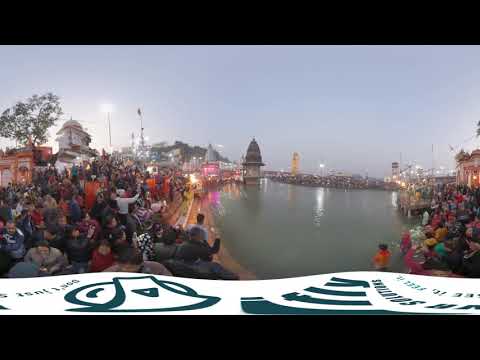The photograph captures an overcast outdoor scene, likely at dusk, centered around a sizable lake or pond surrounded by a dense crowd. The murky, gray-green water is bordered by numerous people, some seated as if on bleachers while others stand, all facing the water. The crowd's appearance and the setting suggest a location outside of the United States, possibly in an Asian town. In the foreground, a white and blue structure bears the word "fly" along with other unreadable text. The backdrop reveals a mix of architectural styles, including a white domed building next to an orange one, and further back a square building topped with a unique beehive shape. The sky above is a dreary gray-blue, lending a muted tone to the overall image. Additionally, an array of lights in pink, white, and reddish hues hint at a celebratory atmosphere. The setting appears bustling and festive, reminiscent of large public gatherings.